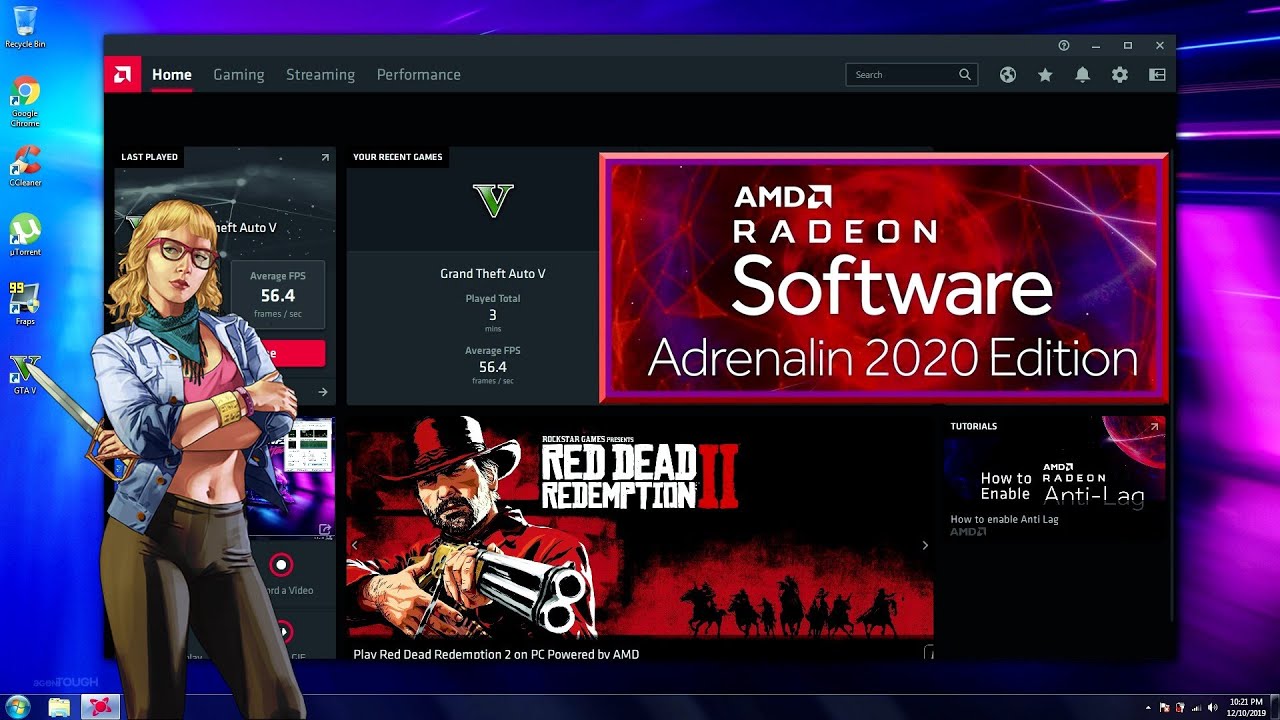The image depicts a computer desktop with a visually striking wallpaper that transitions from various shades of blue on the left to a mix of magenta, navy blue, light blue, and neon colors on the right. On the left side of the desktop, several application icons are visible, including Recycle Bin, Google Chrome, CCleaner, uTorrent, FRAPS, and Grand Theft Auto V (GTAV). The bottom right-hand corner of the screen shows the system clock displaying 10:21 PM and the date as 12/10/2019, with the volume icon indicating that the speakers are active. Next to the clock, the Windows Start menu icon and file explorer shortcut are also visible.

A prominent pop-up window takes center stage on the desktop. The top of the pop-up features a dark gray banner with the word "Home" highlighted in white and underlined in red. To the right of "Home," text in gray reads "Game and Streaming Performance," alongside a search box labeled "Search." Additional icons within the gray banner include a globe, star, bell, and gear, all rendered in gray. Below this banner, the background turns black, showcasing an animated cartoon character brandishing a sword and donning black pants and glasses. The text within the black section reads "Red Dead Redemption 2, Radeon Software Adrenaline 2020 Edition, How to Enable," suggesting a tutorial or guide related to game and streaming performance.